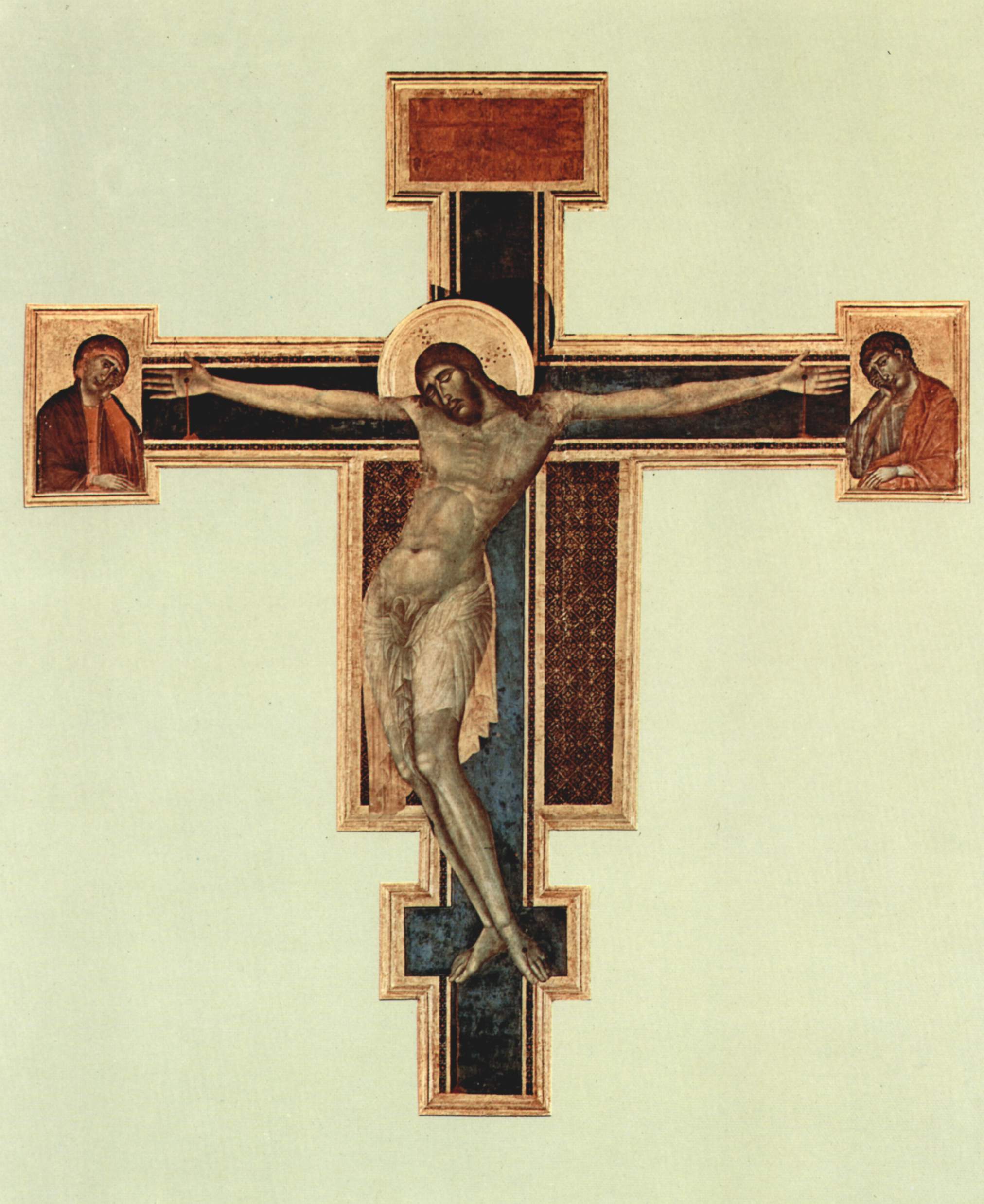The image is a detailed, vertically-oriented picture of an ornate cross that prominently features Jesus Christ at its center. The cross itself is intricately designed with gold borders, and it showcases a mix of teal, burgundy, and black colors in its background, divided in its sections around Christ’s body. Jesus is depicted mostly naked with a cloth draped over his genital area, his head tilted to the left with eyes closed, and a halo-like circle behind his head, adding a sacred aura to the scene.

On either side of Jesus, there are two figures—most likely Mary and Joseph, or other significant religious figures—who are portrayed with their heads resting on their hands, gazing toward Jesus. These figures have their heads aligning towards Christ’s hands, presenting a reverent and contemplative posture.

Above Jesus, the top of the cross is capped in a specific style, and another small crosspiece extends from the bottom. The background behind the cross is a wooden brown, encased further in a larger faded yellow background, adding depth and focus to the central religious imagery. The overall composition lacks any text, focusing entirely on the visual depiction of the crucifixion and surrounding figures.